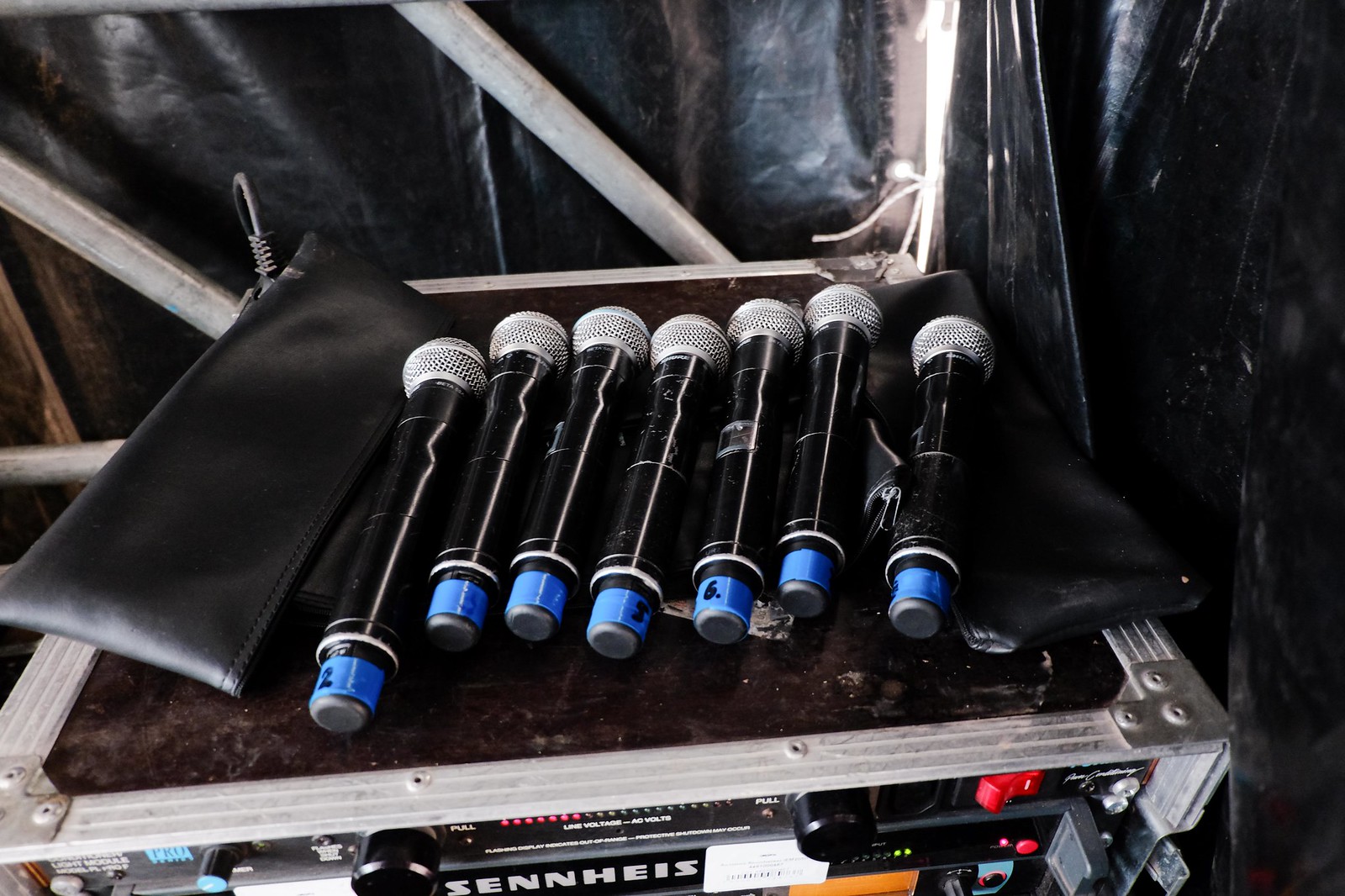This photograph, most likely taken backstage at a live concert, features a detailed setup of electronic gear in a travel case. At the very top, a power conditioner with pull-out round black knobs, which illuminate the front of the rack when extended, is prominently displayed beneath a Sennheiser logo. A row of seven black wireless microphones with silver grills and uniquely numbered using blue electrician's tape and black felt-tip markers is arranged atop the travel case, not a leather tarp. Adjacent to the microphones, a couple of soft bag cases are visible, likely intended for mic storage. The rugged travel case is fortified with riveted corner gussets and metallic reinforced edges that frame the black panels. In the backdrop, black plastic tarps hang alongside diagonal tubes or pipes, hinting at stage construction elements. The overall scene emphasizes a meticulously organized setup ready for a live performance.